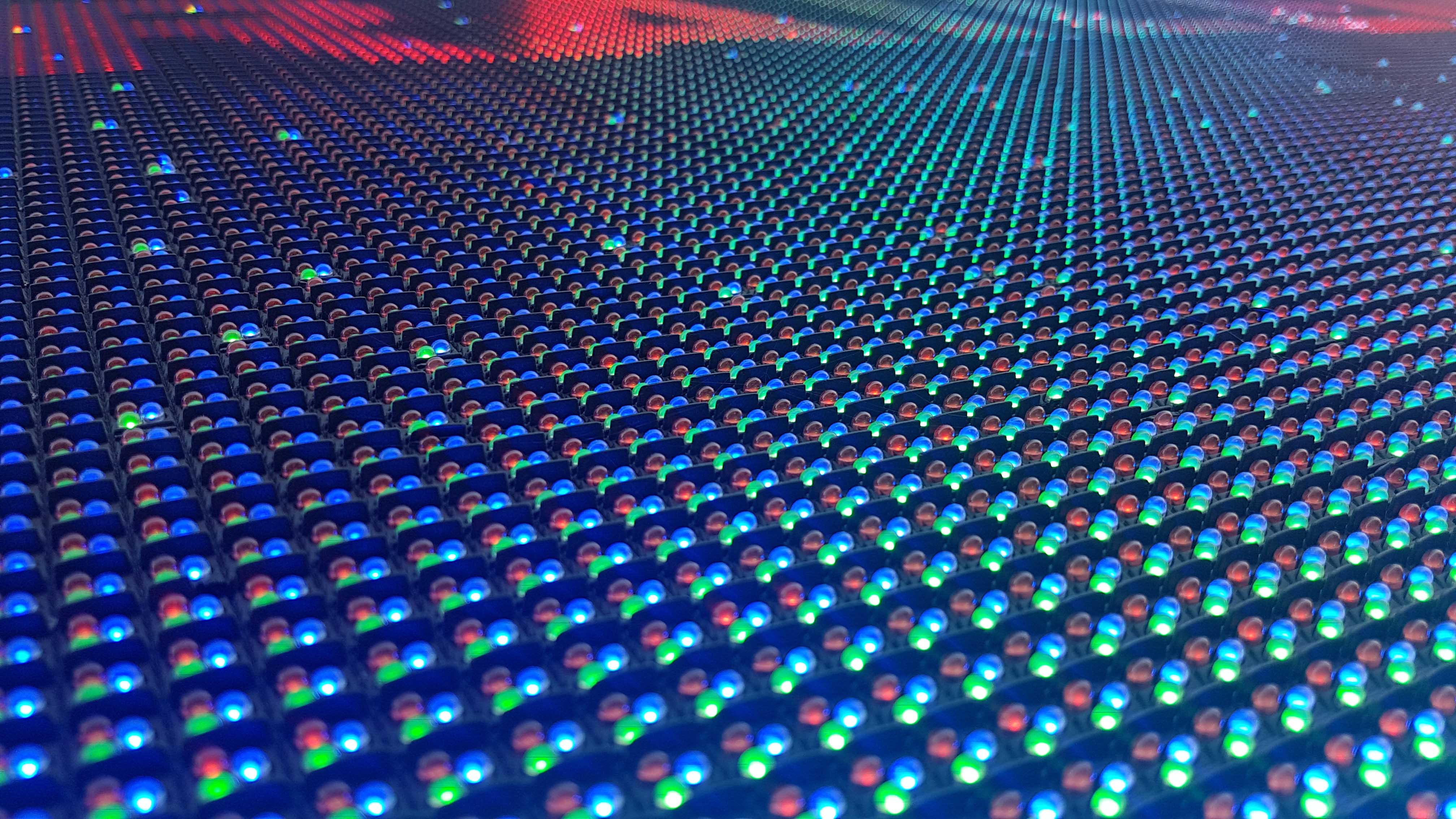The image depicts a photorealistic display, likely of an LED screen, laid flat in a large three-dimensional grid. The grid is composed of numerous small squares, each containing a cluster of red, green, and blue lights that resemble marbles. These lights are arranged in a repetitive pattern, creating an organized, aesthetically pleasing visual. The foreground showcases these clusters prominently, with certain lights appearing to glow more intensely due to a light source casting a glow, particularly a noticeable red light, enhancing sections of the display.

Toward the back and top of the image, the lights shift colors, with some areas dominated by red, spelling out indistinct letters such as an R and an A. This creates a vibrant mosaic of color that transitions smoothly from green and blue at the bottom to red at the top, with occasional highlights of orange, yellow, and violet. The overall appearance is highly detailed and 3D-like, with some lights appearing to stick up more, adding depth to the scene. The background hue varies, contributing to the dynamic and intricate visual effect of the display.